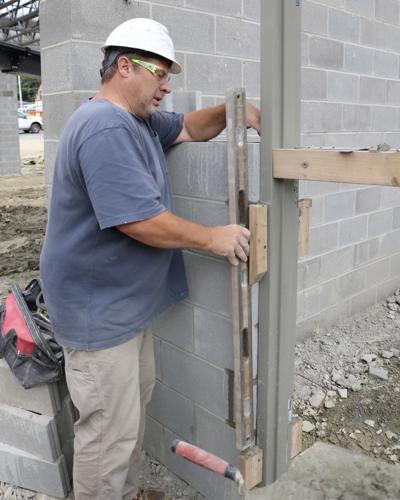The photograph captures a Caucasian contractor, wearing a white hard hat and yellow safety glasses, standing in front of a gray brick wall at an outdoor construction site during the daytime. The man is slightly overweight and is dressed in an oversized blue short sleeve crew neck shirt, tan work pants, and brown boots. He has short hair, possibly brown, and his mouth is slightly open as he focuses on his task.

His left arm rests on the cinder block wall, while his right arm holds a rusted level vertically against the wall, ensuring its alignment. The image shows the man from the ankles up, focusing on his interaction with the wall. To his side, resting on a pile of bricks, is a red tool bag with various tools visible. Scattered across the ground are chips of rock and dirt.

In the background, the wall extends into a corner, and there is a visibly large area of dirt and rocks piled up, hinting at ongoing construction. A working vehicle is parked in the distance, and some scaffolding or structure is partially visible at the edge of the frame, indicating that the contractor is involved in erecting a building or installing fencing.